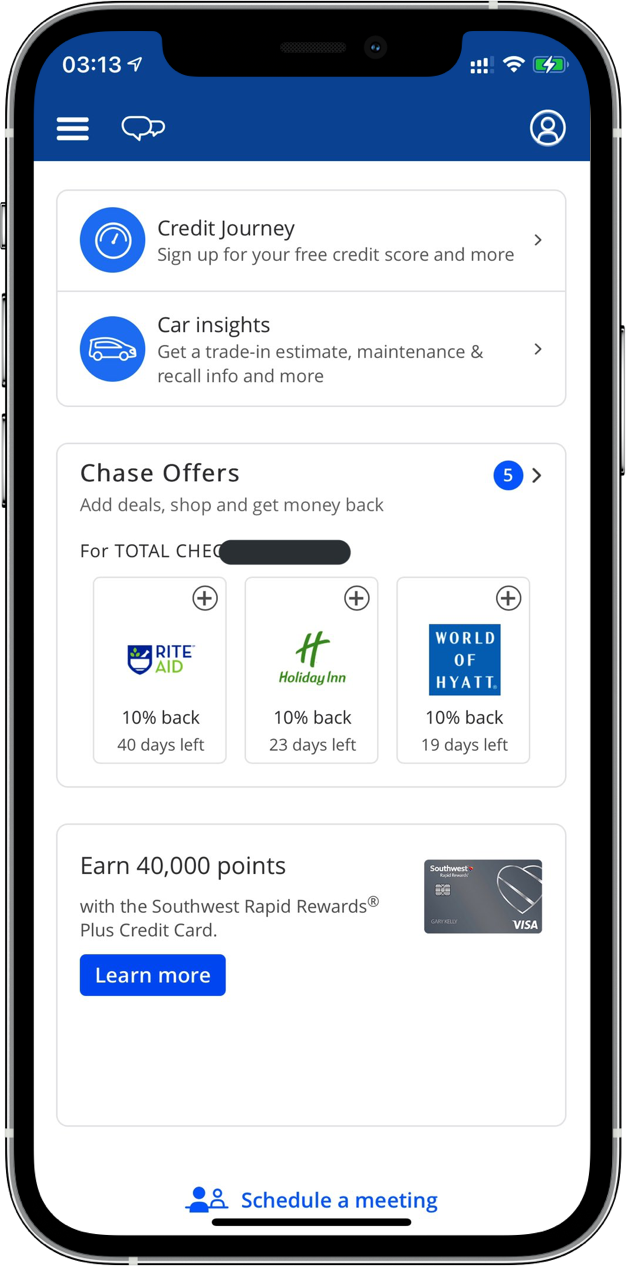The image showcases a cell phone screen displaying a page titled "Credit Journey." At the top, the screen invites users to "Sign up for your free credit score and more." Below this, there is a blue circular icon featuring a car, labeled "Car Insights," which provides options for a trade-in estimate, maintenance and recall information, and more.

Further down the screen, there is a white rectangle bordered with a gray line and rounded corners, labeled "Chase Offers." This section prompts users to "Add deals, shop, and get money back." Some additional text, partially obscured by a black rectangle with rounded ends, seems to mention a "total check."

Three offer options follow: "Rite Aid" with a 10% cashback offer and 40 days left; "Holiday Inn," similarly offering 10% cashback with 23 days left, featuring the Holiday Inn "H" icon; and "World of Hyatt," with a 10% cashback offer and 19 days left.

At the bottom of the screen, users are prompted with an opportunity to "Earn 40,000 points" and a "Learn More" option is available, ending with a "Schedule a Meeting" link.